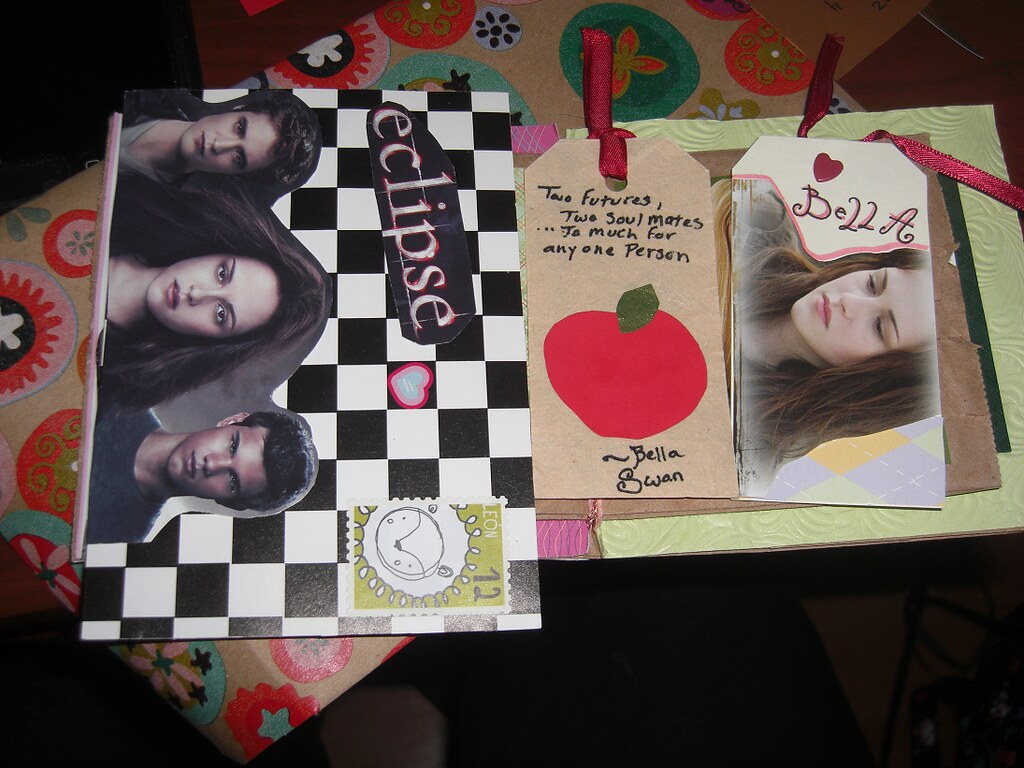The image displays a horizontal rectangular collage of special mementos and craft items, predominantly themed around the Twilight movie series. The base layer consists of wrapping paper, possibly from a previous gift. On top of this paper, there are three notable projects laid out.

On the left side, there's a crafted piece with a black and white checkerboard pattern, prominently featuring the word "Eclipse" at the top. Below the text, a photograph depicts the three main characters from the Twilight series: Bella, Edward, and Jacob. The top right corner of this piece resembles a postcard stamp, colored green with an animal face, and marked with the number 12.

Next to this, occupying the middle section, there's a tag with a meticulously drawn image of an apple (or possibly a tomato) and text that reads: "Two futures, two soulmates, too much for any one person," along with "Bella Swan" inscribed at the bottom.

On the right side of the image lies another tag. This tag features a heart at the top with the name "Bella," and a photograph of Bella Swan, the character from Twilight, gazing down. The woman in the photograph resembles Kirsten Stewart, the actress portraying Bella in the films. This arranged collection of mementos suggests a deliberate and nostalgic effort to commemorate the Twilight series through art and craft.